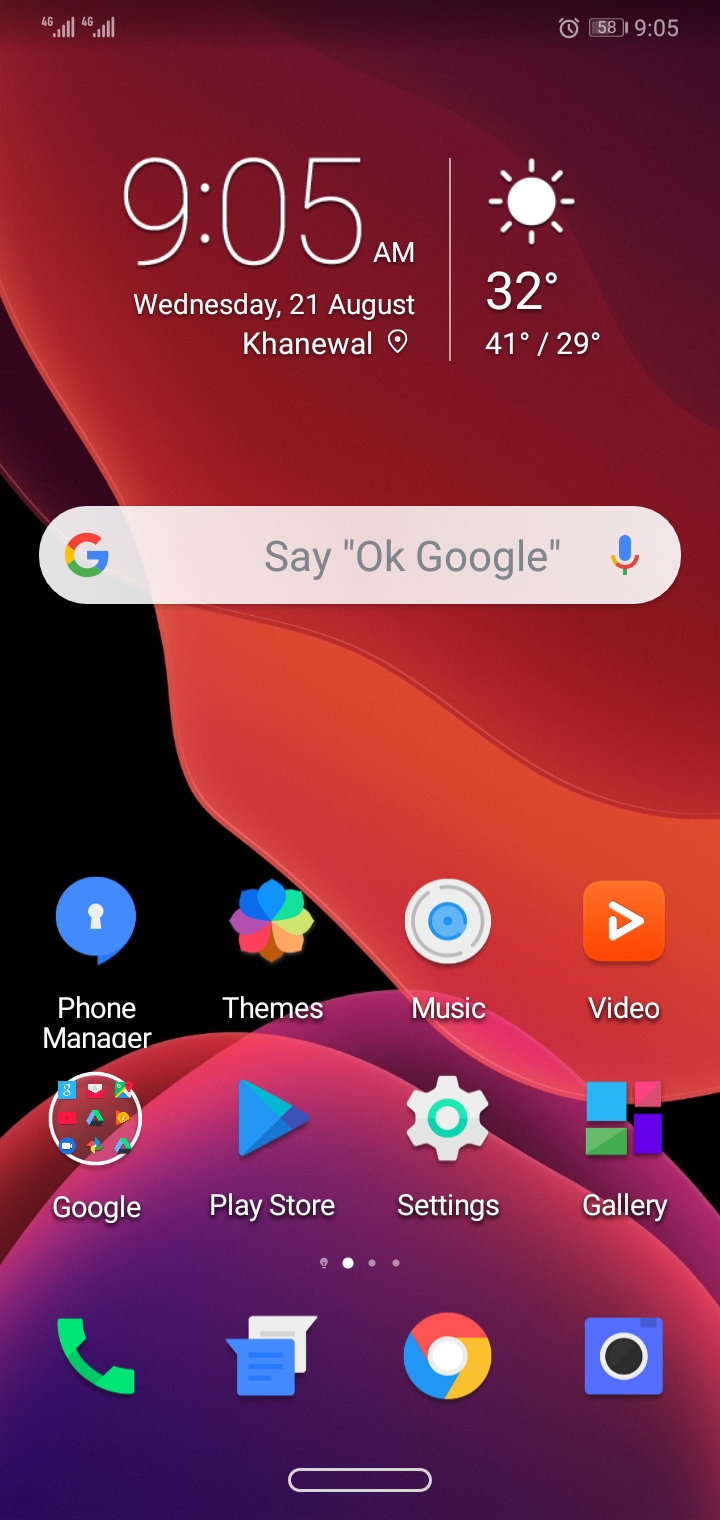The image showcases a smartphone's homepage interface with various details displayed prominently. At the very top, the status bar indicates the time "9:05," accompanied by an alarm clock icon and a battery level at "58%." Below this, the time "9:05 AM" is reiterated in white text, followed by the date "Wednesday, the 21st of August." The location is specified as "Khanewal," labeled "K-H-A-N-E-W-A-L." A weather section appears next, featuring an icon of the sun with the current temperature at "32°C," alongside a daily high of "41°C" and a low of "29°C."

Further down, the Google logo is displayed with a search bar instructing users to "Say OK Google," accompanied by a microphone icon for voice search. The main interface then includes shortcuts to various apps: Phone Manager, Themes, Music, Video, Google, Play Store, Settings, and Gallery. There is also an icon for the phone app, depicted in green, and a chat option, illustrated in blue and white, with opposite-facing arrows.

Additional icons include the Google button and another blue square enclosing a white circle with a black inner circle. The bottom of the screen is marked by a thin line, completing the layout of the homepage.